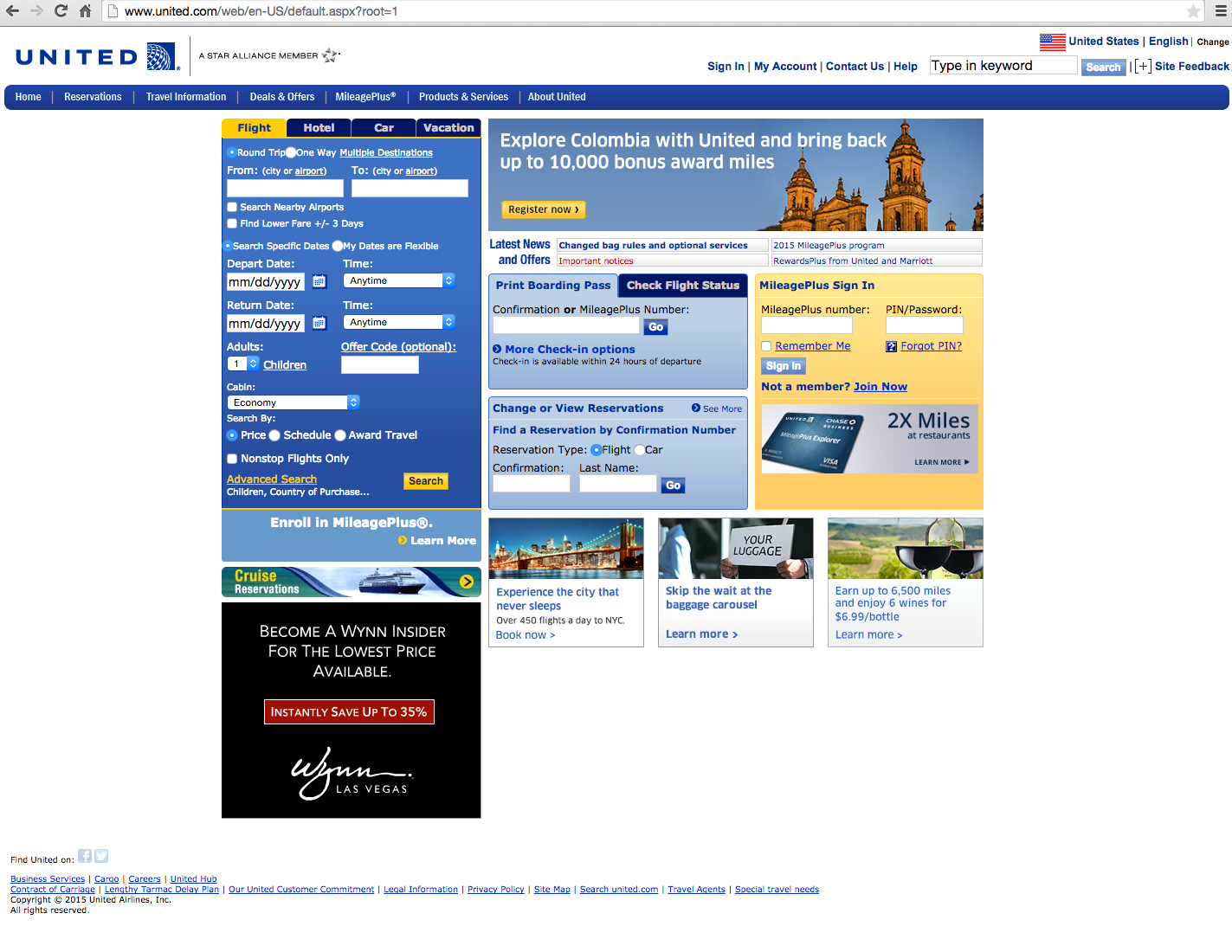This is a detailed snapshot of the United Airlines homepage. At the top, prominently displayed, is the United logo. On the left-hand side, the webpage offers a user-friendly interface to input search parameters for flights, hotels, car rentals, or vacation packages. Users can enter specific details such as travel dates, the number of passengers, and the desired class category. To the right, there are additional fields that allow for a MileagePlus sign-in, options to view or print a current boarding pass, and other related functionalities. Along the bottom of the page, there are three tiled menus, although the text within these tiles is too small to read clearly. The overall layout is designed to provide seamless navigation and a comprehensive booking experience.